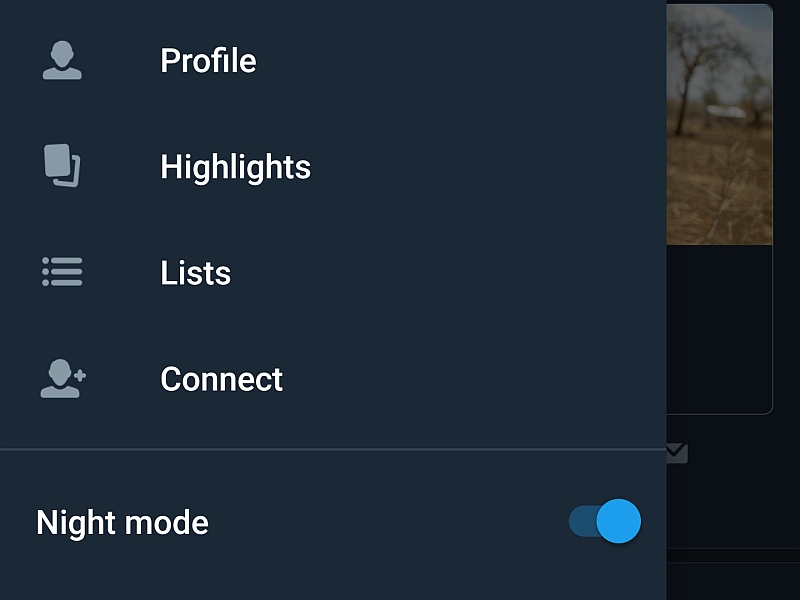The image depicts a web page with a drop-down overlay, revealing only a margin of the underlying page. The background of the main screen appears predominantly black, while the upper portion showcases a photo. The drop-down section, set against a navy blue background, features several user interface elements. 

At the top of this navy blue screen is the word "Profile" in white font, accompanied by a head-and-shoulders icon. Below this, the word "Highlights" is similarly displayed in white. Adjacent to it are two rectangles, one filled and the other outlined in gray. Following this, the word "Lists" is displayed in white text, next to which are three horizontal lines each accompanied by a dot on the left side. Lastly, the word "Connect" appears in white, beside an icon of a person with a plus sign near the head.

Underneath the options, a thin purple line runs horizontally across the screen. Below this line is the "Night Mode" option, marked by white text. This feature is indicated to be active as highlighted by a turquoise blue button to its right.